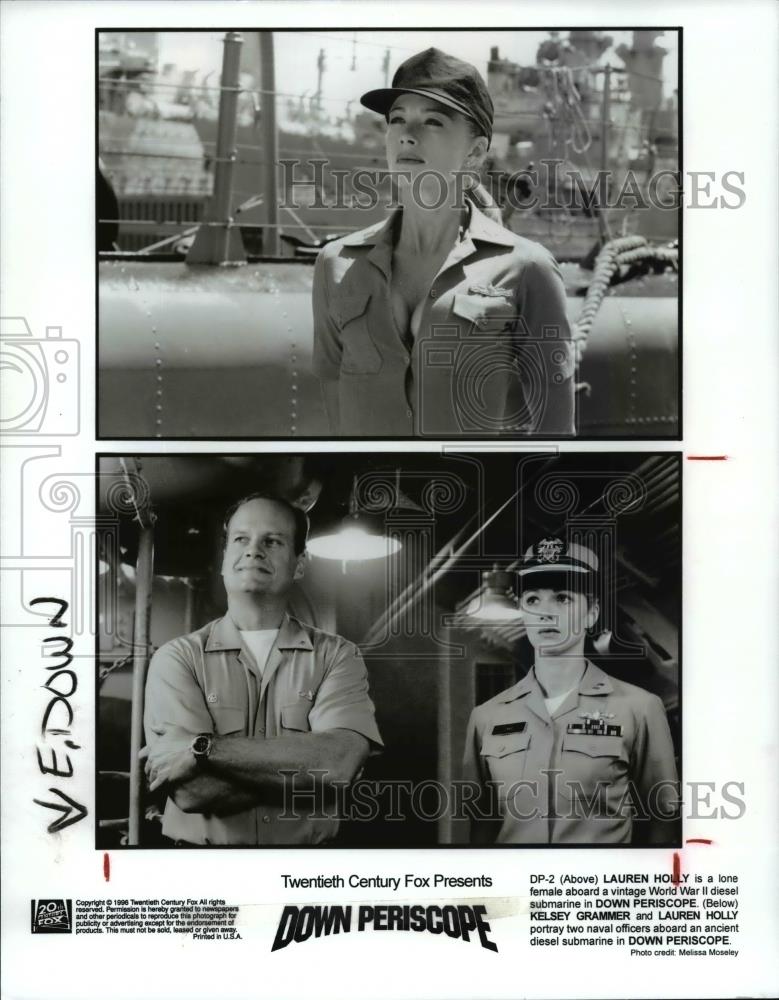This is a black-and-white movie poster for 20th Century Fox's "Down Periscope," featuring a watermark that reads "Historic Images" prominently at the top and bottom. The poster showcases two distinct black-and-white photographs. At the top, Lauren Holly, dressed in a military outfit and wearing a hat, gazes into the distance with a serious expression. Below, Lauren Holly stands next to Kelsey Grammer; he is smiling slightly with his arms crossed, revealing a watch on his wrist. Both are depicted as naval officers aboard a vintage World War II diesel submarine. The caption at the bottom confirms that Lauren Holly is the lone female officer on the submarine, highlighting the dynamic between these two characters. The text at the bottom reads: "20th Century Fox presents Down Periscope."